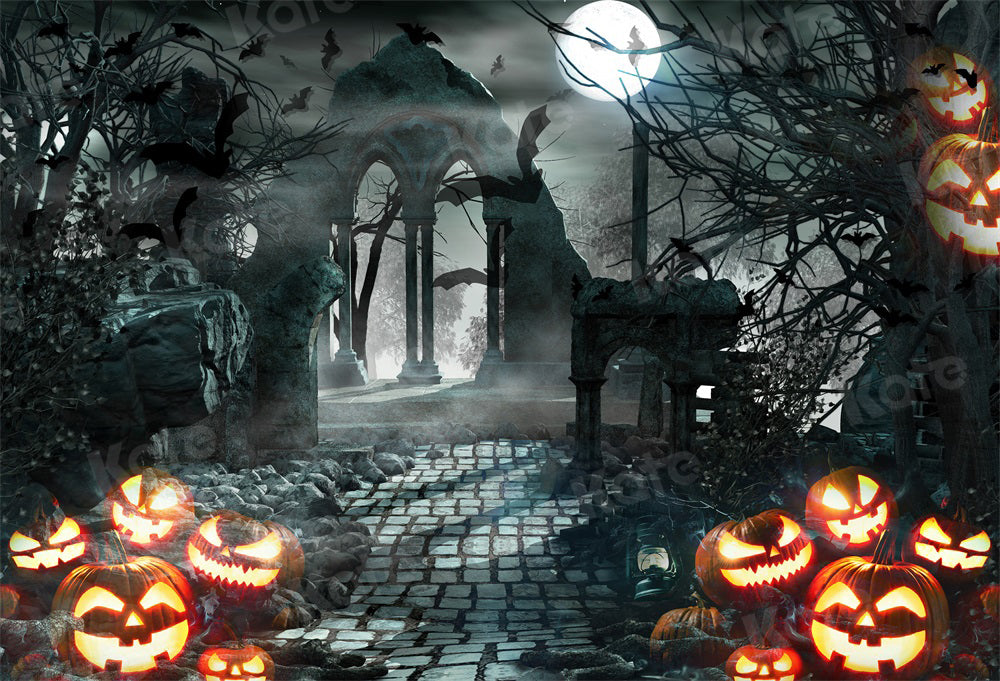In this eerie and atmospheric Halloween-themed artwork, a full moon casts a ghostly light over a haunting scene. The sky is dark and black, punctuated by bats flying through the night air. At the center of the image, a triangular stone archway with two openings, separated by thin columns, stands prominently. Leading down from this archway are stone steps that descent to a cobblestone path, forming a compass shape, which extends towards the foreground.

On either side of this path, in the bottom left and right corners of the image, several orange jack-o-lanterns with carved faces display a variety of wicked smiles and menacing expressions. Additional, somewhat transparent jack-o-lanterns hover ominously in the top right corner. Adjacent to these pumpkins are barren trees, their twisted branches adding to the overall sense of decay and desolation.

The scene is enveloped in a thick, rolling fog that enhances the spooky ambiance, making it an ideal backdrop for a haunted house or Halloween celebration. While the details of a copyright mark are visible, they are too faint to read clearly. The entire illustration evokes a chilling, yet intriguing, Halloween horror atmosphere.